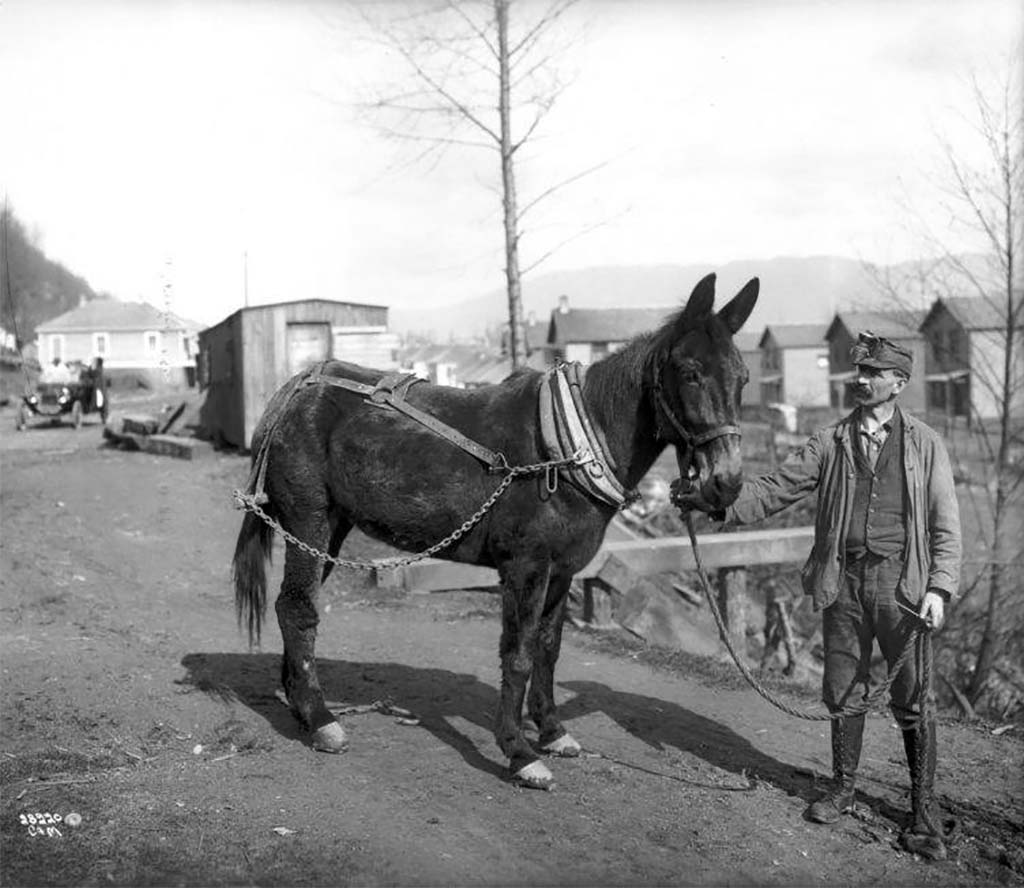The vintage black-and-white photograph likely dates back to the late 19th or early 20th century and depicts a working man standing beside a donkey on a roadway. The sky and a small community of houses and buildings form the backdrop, with a car visible to the left, suggestive of the early 20th century. The man is dressed in knee-high boots, trousers tucked into the boots, a long-sleeved shirt, a vest, a lighter jacket, a tie, and a cap, indicating he is likely a laborer or farmer. The donkey, facing right towards the man, is equipped with a harness around its neck and back, a rein attached to a thick rope held by the man, and a chain connected to a pole behind its tail. The background features a bare tree, hinting at cold weather, and the ground appears to be snow-free. The photograph is marked “28220CNM” in the bottom left-hand corner.